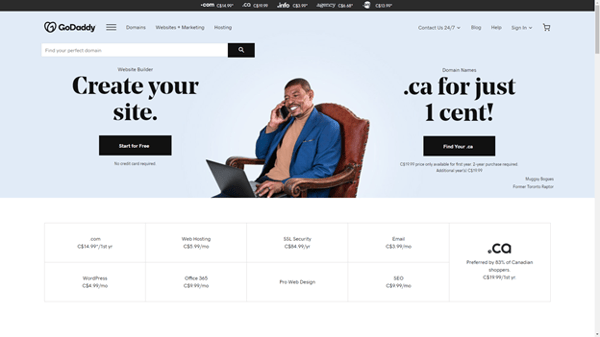This is an illustrative screenshot taken from the website of GoDaddy.com, a prominent web hosting company, showcasing their various services and offerings. The image is wider than it is tall, indicating it was likely captured from a computer screen. 

At the very top, there's a noticeable black rectangular bar, and below it, slightly blurred, are several browser tabs. Directly beneath this, lies a prominent blue rectangle displaying the GoDaddy logo alongside their tagline "Create your site." 

Underneath the blue banner is another black rectangle featuring white text that reads "Start for free." The focal point of the visual content is an individual seated in a chair. In the person’s right hand, they are holding a cell phone, while their left hand is actively positioned on the trackpad of a laptop resting on their lap.

To the right of this individual, text promotes domain names, specifically ".ca" domain names for just one cent, suggesting a focus on the Canadian market. Some of the text that follows, "Find your," is slightly too blurry to be legible.

At the bottom of the screenshot, there is a table composed of nine sections arranged in two rows of four columns, with an adjacent rectangle on the right spanning both rows. This rectangle prominently displays ".ca" and additional text that aligns with GoDaddy's domain pricing options. Each of these segments lists different plans and prices, indicating the various packages that GoDaddy offers for domain registration and site creation. This visual representation implies that visitors to the site can easily create their website and register a domain name simultaneously.